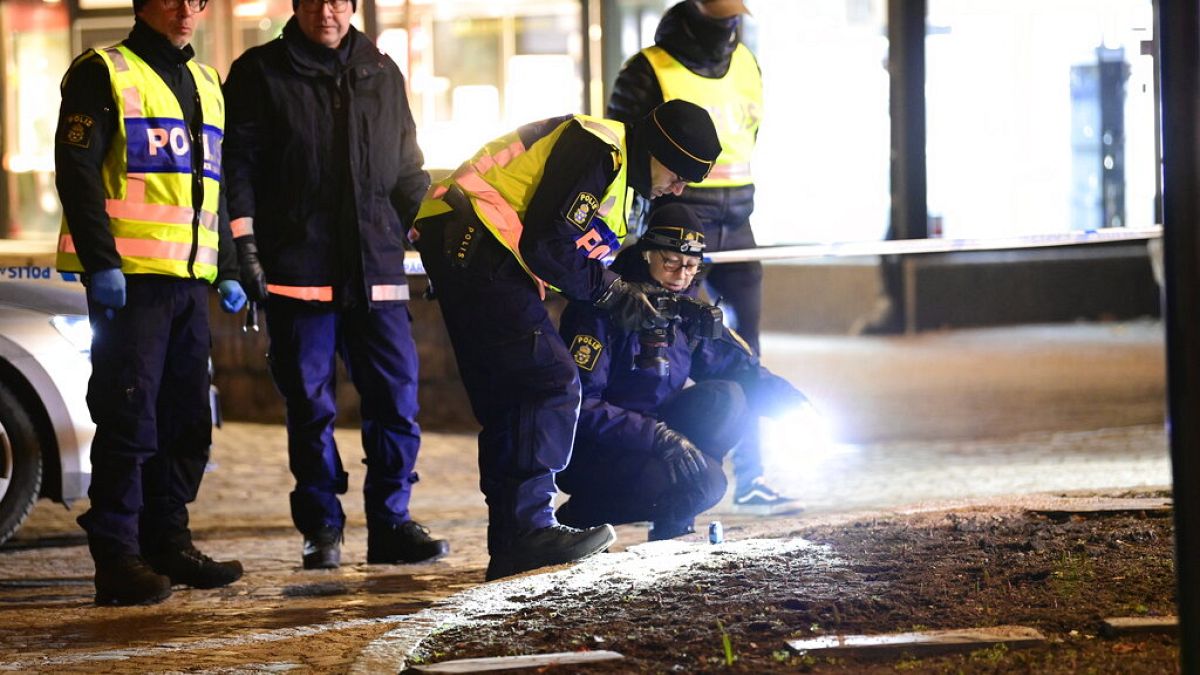This nighttime scene depicts a group of five police officers conducting an investigation on a city street. Central to the image, a police officer, possibly a woman, is crouching on the dirt, wearing glasses, a blue jacket, and blue cargo pants. She is shining a flashlight over an area on the ground, while another officer next to her, wearing a black knit cap, a yellow vest with a blue stripe, and blue pants, is leaning over with a camera, seemingly capturing evidence. To their left, two men stand side by side; one is dressed in a black jacket and jeans, while the other, a police officer, sports a yellow vest marked "POLICE" and blue gloves. Both have their foreheads cut off at the top edge of the image. Behind them, partially visible, is the front of a police car and police tape stretching from left to right, cordoning off the scene. In the background, beyond the tape, another officer stands in a yellow vest, with illuminated storefronts providing a backdrop to the focused activity in the foreground.